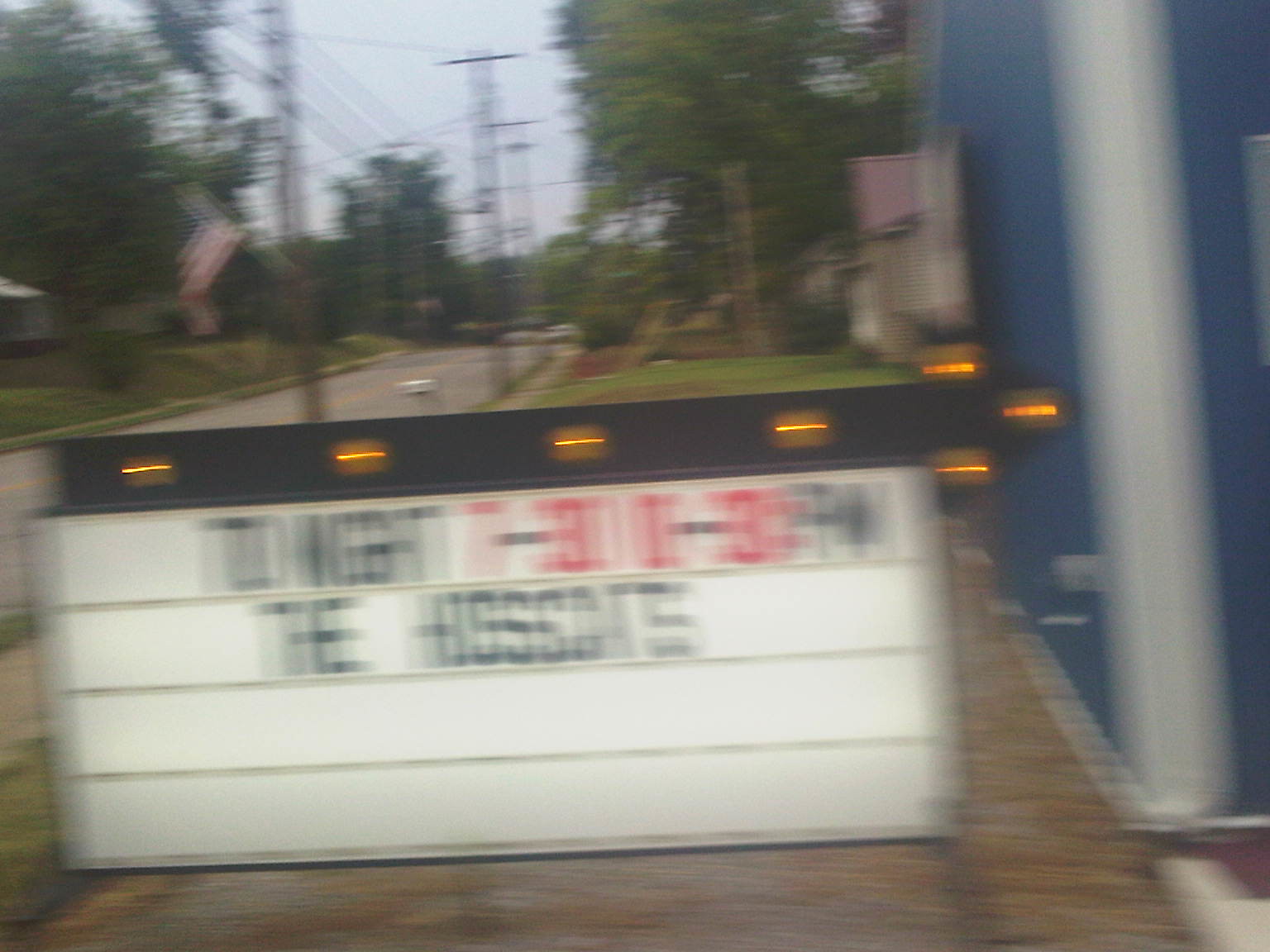The image features a weathered, outdoor business sign with a white background and metal frame. The sign is designed with four rows of slots for inserting interchangeable letters or characters, which are typically used to display various messages. The metal slots create indents where the letters are slid in. 

The top row of the sign has a somewhat legible message that reads, "Tonight 7-8 PM The Hogs," although the last part is blurry and unclear due to the low quality of the photograph. The overall condition of the sign appears aged and slightly worn, indicative of its prolonged exposure to the elements. The image captures a slice of everyday community life, emphasizing the utilitarian nature of such signs in relaying local events or business announcements.